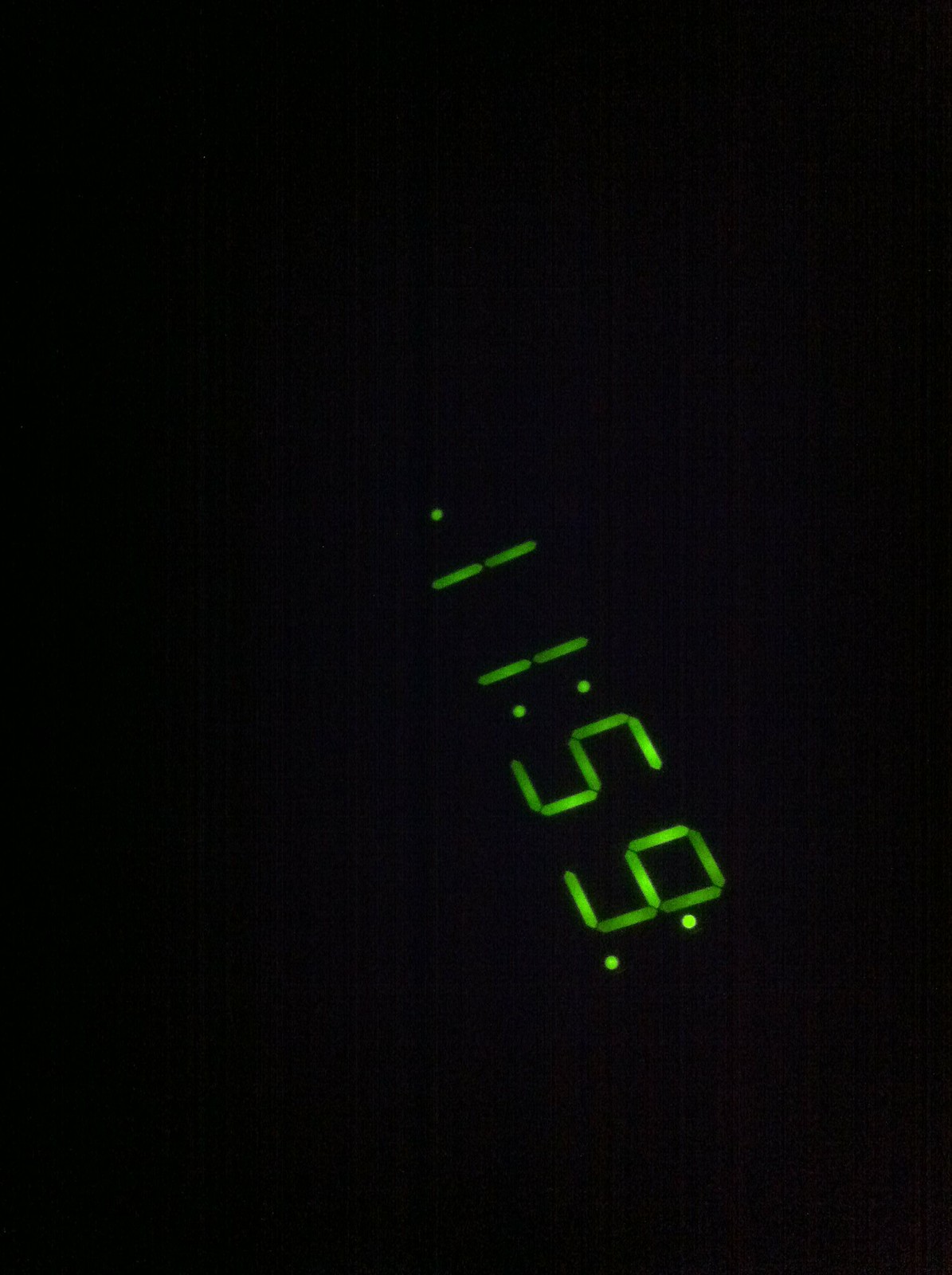The image features a glowing green digital clock display set against a completely black background. The time, "11:59," is arranged diagonally from the top left to the bottom right. The sequence begins with a single dot at the top left, followed by the numerals "1" and "1", two dots in the middle, a "5", and a "9", and ends with two more dots. The entire background is a deep, uninterrupted black, providing a stark contrast that highlights the vivid, neon-like numbers.